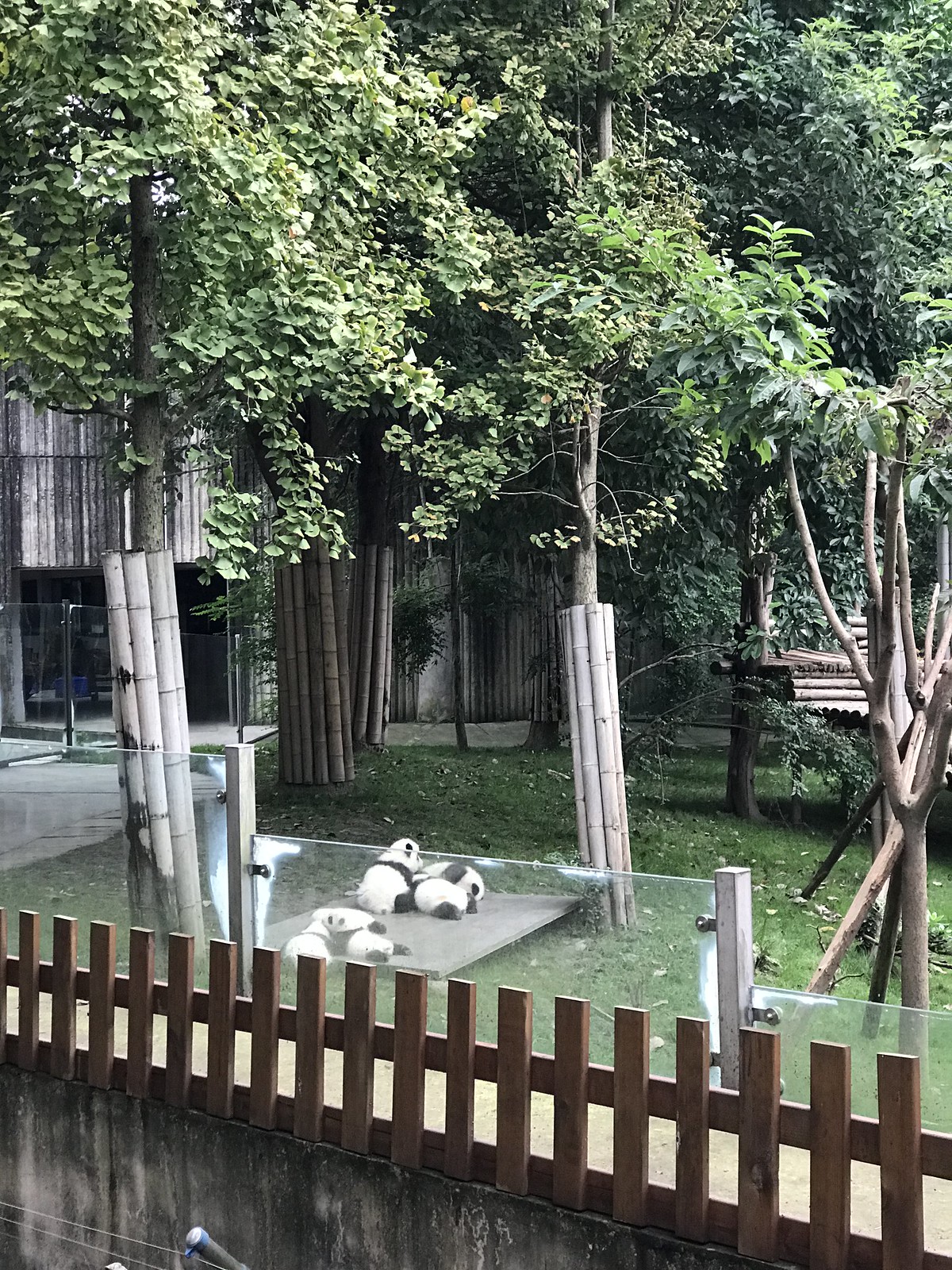The image depicts a panda enclosure at a zoo, taken during the daytime. The setting is an outdoor area surrounded by a concrete wall topped with a white picket fence and clear, transparent panels. Within this enclosure, five pandas can be seen lounging on a platform positioned between two trees on a grassy field. The pandas are grouped, with three on one side of the platform and two on the other, appearing to lie on top of each other. The pandas exhibit typical markings, with white bodies and black patches around their small eyes, though their faces are not prominently visible. Encircling the tree trunks are protective rings of dried bamboo, presumably to prevent the pandas from damaging the bark. The grassy area is punctuated by scattered trees, and in the background, there are thicker tree clusters, additional clear panels, and a concrete fence or part of a building. A staircase and a walking path are visible, indicating that visitors can walk around the enclosure and observe the pandas.